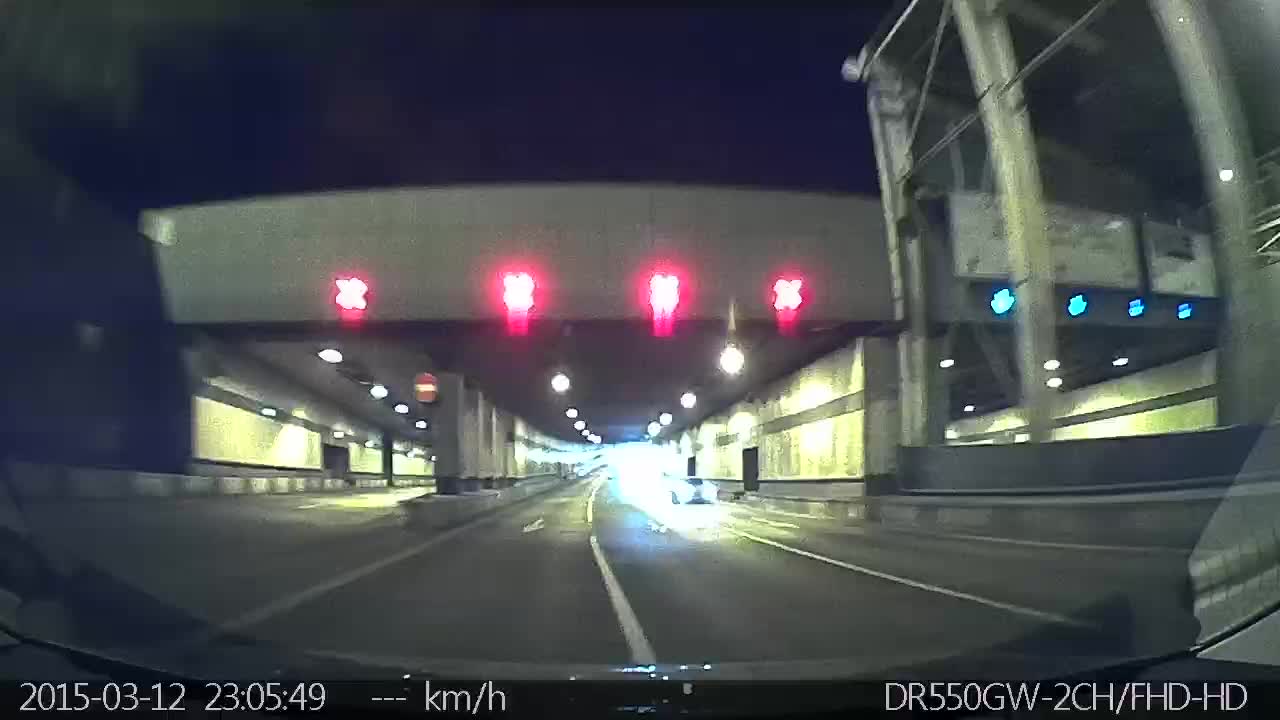This nighttime photograph appears to be taken from behind the windshield of a motorcycle on a highway. The perspective shows the vehicle exiting a highway tunnel or toll booth area. In the foreground, there are multiple lanes marked by a concrete overhang. Each lane has a red light above it, signaling that entry is prohibited. Meanwhile, the road markings below feature arrows pointing outward, reinforcing the direction of travel out of the tunnel. To the right, another set of lanes, also under a concrete overhang, is visible. These lanes display green arrows, indicating that they are open for entry. The juxtaposition of red and green signals creates a clear narrative of exiting and entering traffic zones in this urban nightscape.